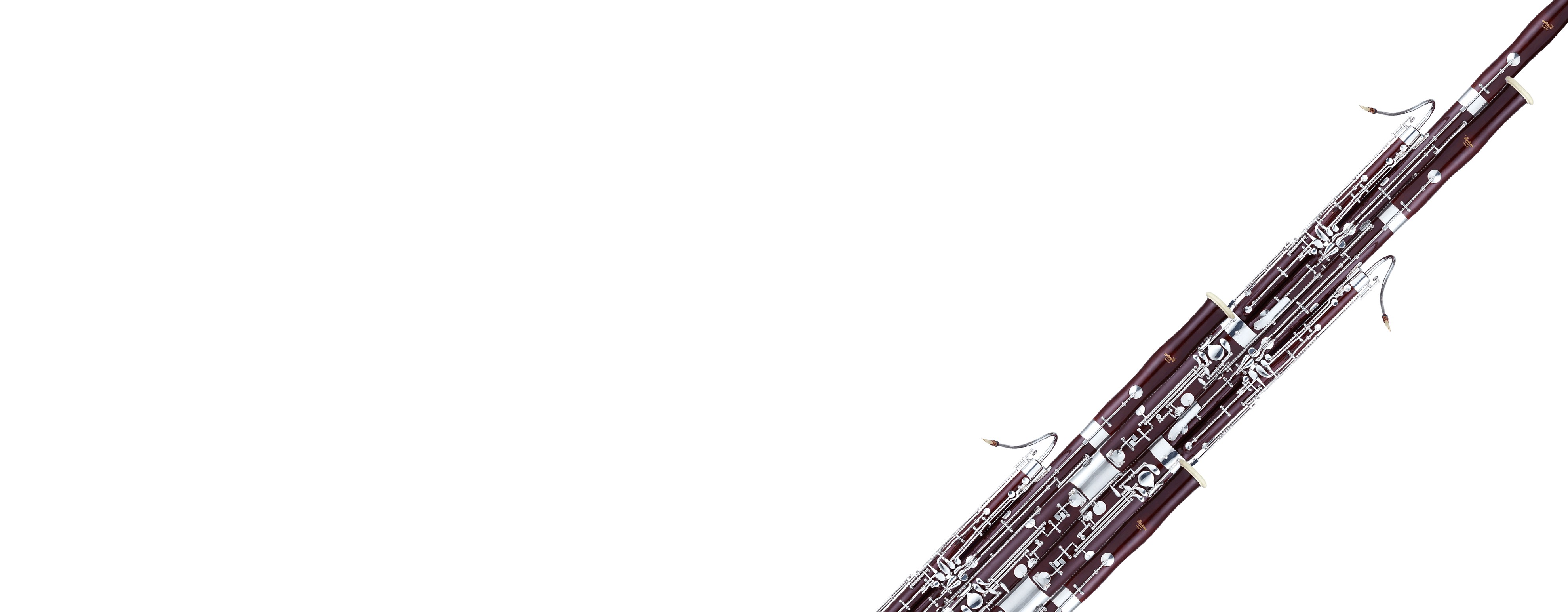This photograph features a diagonally oriented woodwind musical instrument, extending from the bottom left corner to the top right corner of the frame, against a white background. The instrument is predominantly a maroonish brown color, accentuated with numerous silver details. Seven rods of varying lengths protrude from the main body, each adorned with different ends—some flat, others equipped with small mouthpieces or silver attachments similar to those found on flutes and clarinets. These attachments include several silver curving lines, grommets, and intricate finger buttons used to control the instrument's notes. The combined elements create a complex and visually appealing design, with the contrasting dark brown (or possibly black) and silver finish contributing to its detailed appearance.